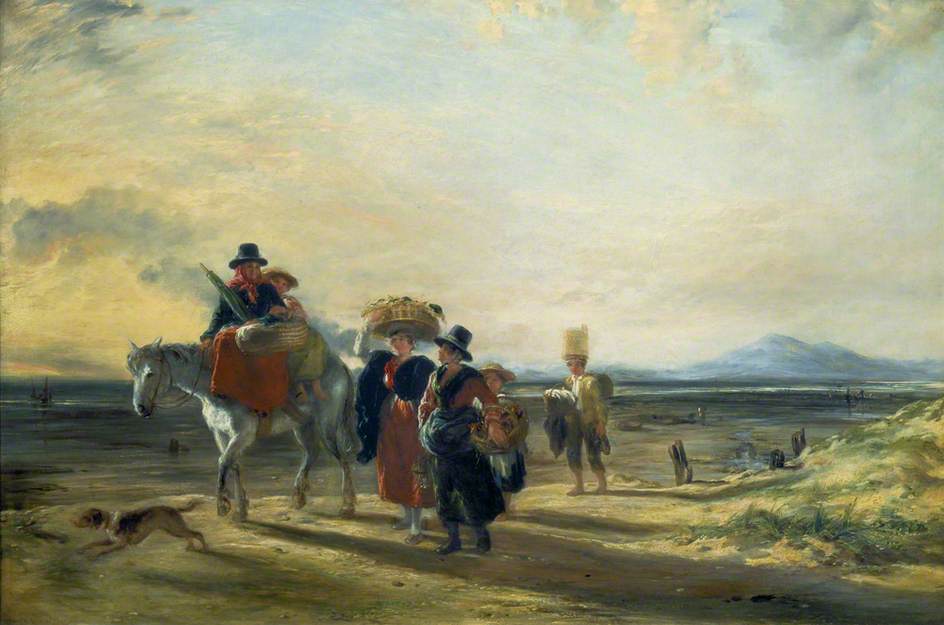This horizontally aligned rectangular painting on a textured canvas features a vast and detailed scene. The upper part of the painting showcases a cloudy sky with blue tones at the very top. Grayish white clouds dominate the upper left corner, while the upper right corner has varying shapes of puffier white and gray clouds. Moving down toward the center, elongated rows of whitish-gray clouds stretch across the sky. The middle to the bottom part of the painting depicts a largely barren, dirt-covered expanse with visible rocks and sparse green grass. In the background, there are faint silhouettes of grayish mountains, suggesting an expansive horizon.

The main focus is a white horse walking towards the left, with two people riding on it. The woman in front, wearing a black hat, red scarf, black top, and long dress, holds an orange bag and possibly a green umbrella. Behind her is another rider with a brown hat. Walking alongside the horse is a small brown dog, running in the same direction.

On the ground, four people interact with the riders. A woman in an ornate black and orange dress balances a large basket with a floral arrangement on her head, while another person next to her, possibly a man, wears a black hat and an orange and black outfit. Behind them are two more individuals; one is a woman in a black skirt and straw hat, partially obscured by her basket, and another appears to be a man with a tall, distinct headdress, holding a blanket and walking barefoot.

The composition suggests a family or a group traveling through a barren desert at sunset, characterized by the long shadows and unique light emanating from one side, accentuating the textured landscape and serene sky.